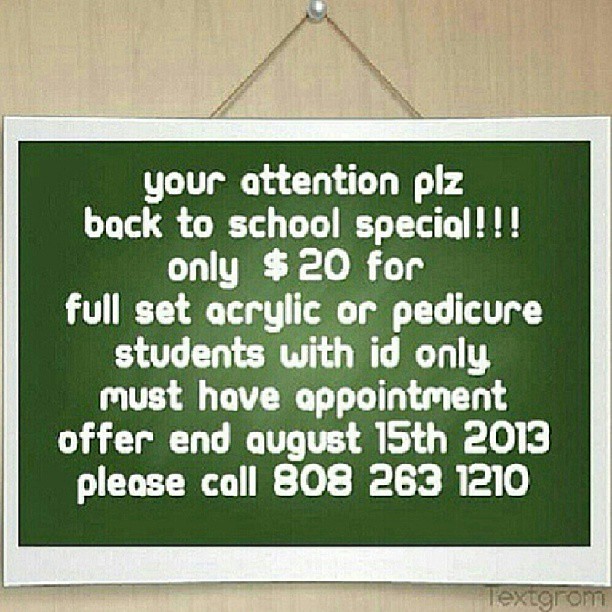The image shows a sign hanging on a pearl-like thumbtack, affixed to a light wood-colored surface that resembles a wooden wall or door. The sign itself is square, with a green background that features a radial gradient from light green in the center to dark green at the edges, bordered by a white frame. Suspended by a piece of string, the sign's text is in white and reads: "Your attention, PLZ. Back to school special!!! Only $20 for full set acrylic or pedicure. Students with ID only. Must have appointment. Offer ends August 15, 2013. Please call 808-263-1210." The bottom right corner of the sign features faint light gray text that says "TEXTGRAM." The digital nature of the image is apparent due to its pixelated quality.